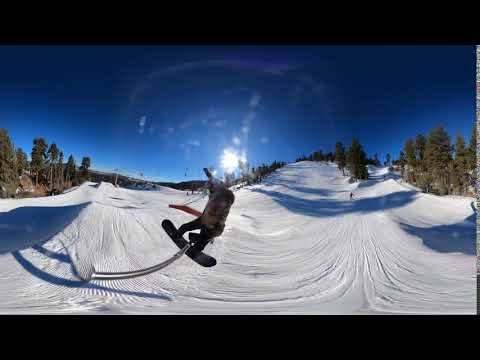The image depicts a man snowboarding on a snowy slope, riding a dark-colored snowboard. He is dressed in black pants and a brown jacket. The snow-covered landscape is flanked by tall, somewhat dull green pine trees with sparse snow on them. The clear blue sky above is lightly distorted, possibly due to a fisheye lens effect, making the scene appear slightly circular and magnified in the center. The sun peeks just over the horizon, creating lens flare effects and casting shadows across the slope, possibly from the trees or clouds. In the distance, to the right, another small figure can be seen descending the hill. The overall setting resembles a ski resort with ramps and the atmospheric distortions, emphasizing the central snowboarder's dynamic movement, possibly airborne and holding a selfie stick.